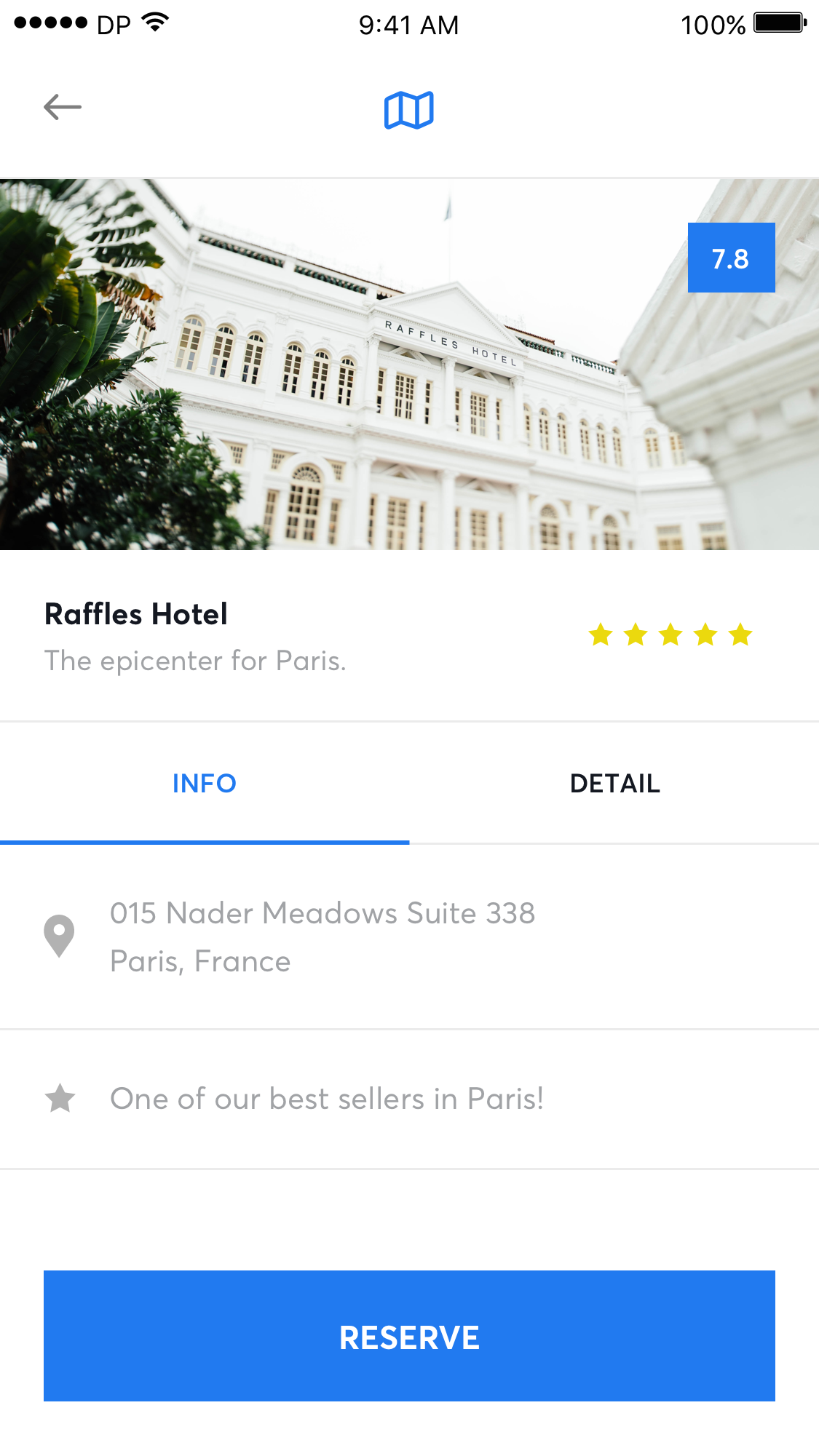The screenshot, taken on an Apple device, captures a hotel reservation app interface. At the very top, the iPhone status bar displays the carrier information, Wi-Fi signal, the time (9:41 AM), and a fully charged battery (100%). 

Occupying the main section of the screenshot is a large image of the hotel being viewed. In the top right corner of the hotel image, a small numeral "7.8" is visible, though its significance isn't clarified. Below the hotel image, the hotel's name, "Raffles Hotel," and a brief description, "The Epicenter for Paris," are prominently displayed. To the right of the hotel name and description, a 5-star rating (5 out of 5 stars) is shown, indicating high user approval.

Underneath this segment, the app displays several informational tabs, with the "Info" tab currently active. This section details the location as "015 Nader Meadows Suite 338, Paris, France," followed by a note mentioning the hotel's popularity: "One of our best sellers in Paris." 

At the bottom of the screenshot, a large blue "Reserve" button is prominently positioned, inviting users to book their stay at the Raffles Hotel.